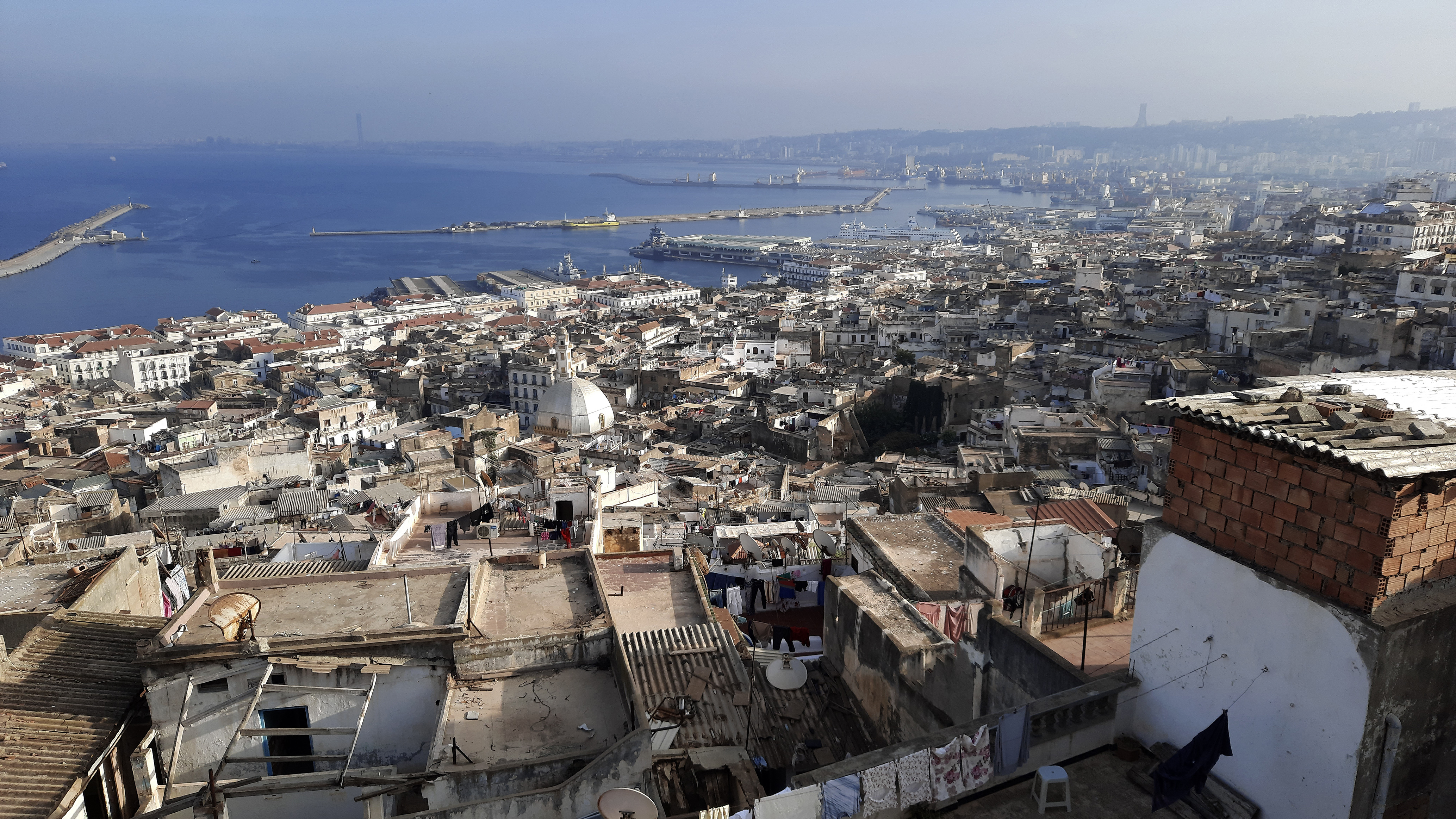The image showcases an expansive aerial view of a seaside community, characterized by a mix of residential and commercial buildings. In the foreground, various structures predominantly built with brick and featuring white facades create a vivid contrast. Among them, some appear dilapidated with metal roofs secured by rocks or miscellaneous materials, and clotheslines stretched across rooftops. The cityscape, which includes both modest homes and larger edifices closer to the water, seems to reflect a lower economic status. Extending towards the coast, the background reveals a serene bay with strikingly blue waters, accompanied by strips of land jutting into the sea. The horizon is veiled in a hazy, foggy light, suggesting a misty day. Despite the somewhat indistinguishable country of origin, clues like the presence of harbor facilities, potential bridges, docks, and the industrial appearance of some structures hint at a potentially Mexican town. Overall, the image portrays a complex, multifaceted community that is tightly knit against a picturesque coastal backdrop.